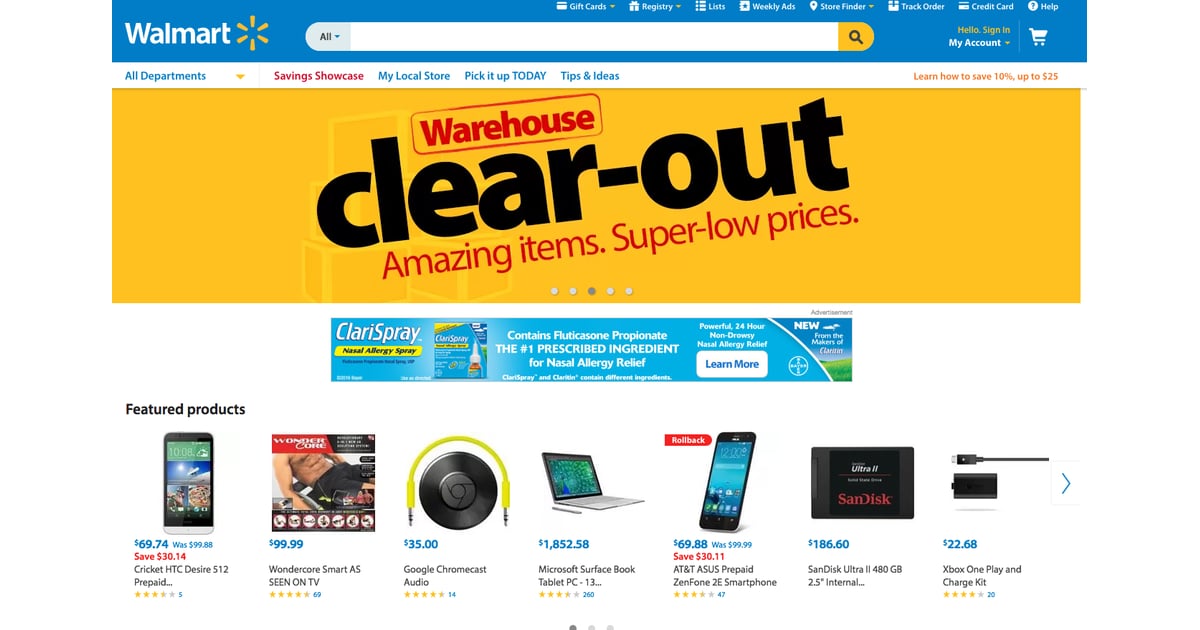**Detailed Caption:**

This is a comprehensive screenshot from Walmart's website. The interface is thoughtfully organized, starting with a prominent blue bar at the top. Located on the upper left-hand side of this bar, the Walmart logo is displayed in clean white lettering, paired with a distinctive yellow sunburst design. Dominating the central portion of the blue bar is an elongated white search bar. On the left side of the search bar, there's an "All" dropdown menu. Meanwhile, the right side of the search bar features a yellow area containing a magnifying glass icon for easy search initiation.

Above this primary navigation area, the topmost section offers several categories: "Categories," "Gift Cards," "Registry," "Lists," "Weekly Ad," "Store Finder," "Track Order," "Credit Card," and "Help." Situated just below, it greets visitors with "Hello, Sign In," "My Account," and a shopping cart icon.

Beneath the blue bar, a secondary white navigation bar provides additional options: "All Departments" with a dropdown menu, "Savings Showcase," "Read My Local Store," "Pick It Up Today," "Tips and Ideas," and a promotional area on the right stating, "Learn how to save 10% up to $25."

Taking center stage, a large yellow rectangular banner prominently announces a "Warehouse Clear-out" in bold black letters, followed by "Amazing items, super low prices" in vivid red text.

Showcased below the promotional banner, a section titled "Featured Products" includes seven highlighted items:

1. **Cricket HTC Desire S12 Prepaid Cell Phone:** Priced at $69.74 (originally $99.88), with a blue label indicating a $30.14 savings in red text. The product description abbreviates, with a visible rating of approximately 3.5 out of 5 stars, based on five reviews.
   
2. **Exercise Machine:** Displaying the midsection of a lean white man with six-pack abs wearing black shorts. Multiple small circles below show additional images of the same item, accompanied by its price, description, and star rating.

3. **Google Chromecast Audio Gadget:** Featuring a yellow cord with two plugs and a central black disc, this audio device is priced at $35 with ratings available.

4. **Microsoft Tablet:** Showcasing a beautiful peacock with its feathers fully fanned out on the screen. The display includes the tablet’s name and star rating.

5. **AT&T Cell Phone:** Details visible, accompanied by rating information.

6. **SanDisk Product:** Specifically, a 480-gigabyte storage device, including ratings and descriptions.

7. **Xbox Charge Kit:** Briefly described with visual representation and star rating.

Overall, this screenshot meticulously captures the structure and offerings of Walmart's website, effectively illustrating the user interface and featured products.